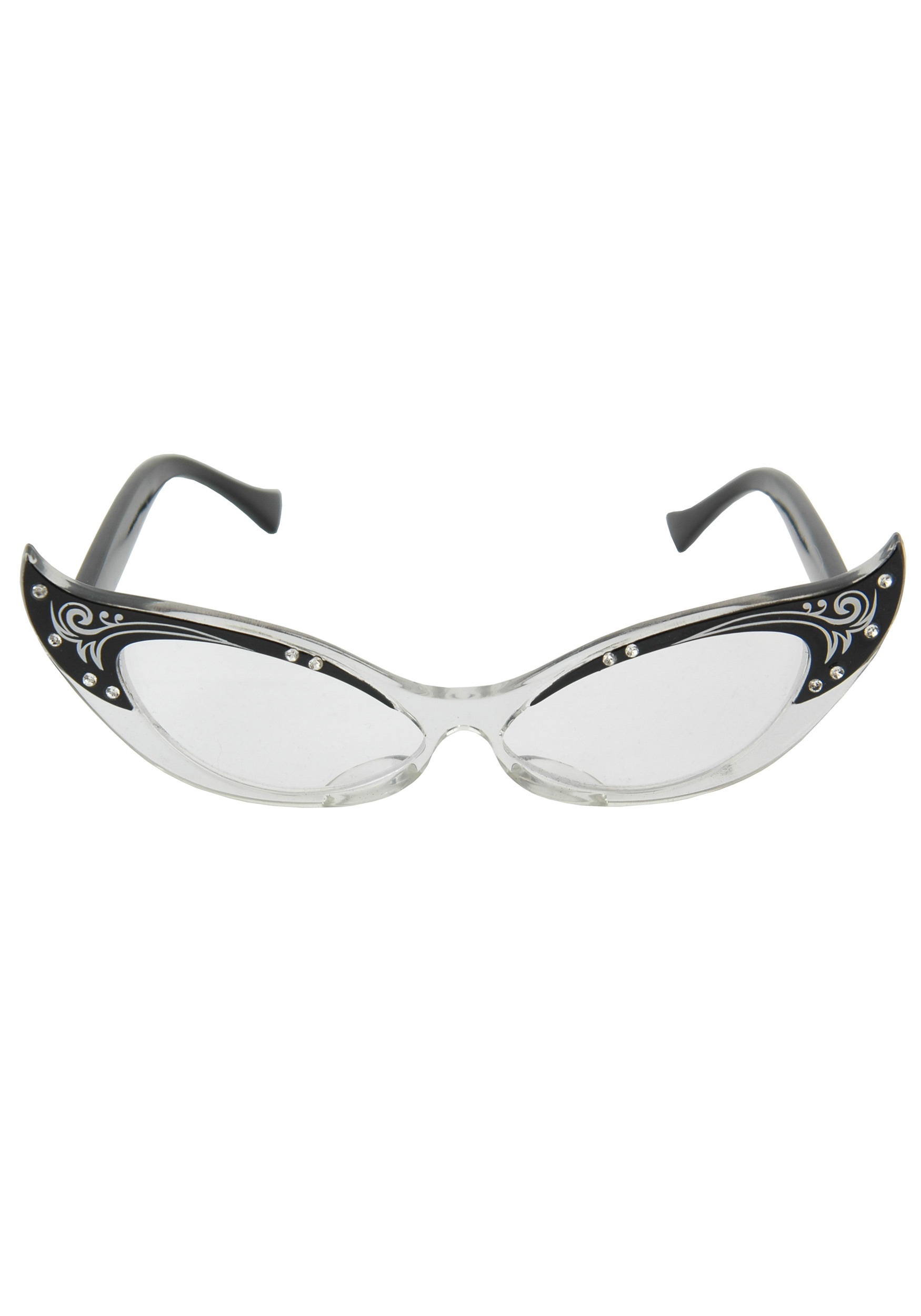This image features a detailed, front-facing photograph of a pair of unique cat-eye eyeglasses set against a white background. The eyeglasses exhibit an elegant design with clear lucite frames and striking black top edges. Each black section is intricately adorned with a captivating black and white swirl pattern, complemented by etched designs and embellished with four tiny, clear crystals on each side and two in the center above each lens. The lenses themselves are light gray, harmonizing with the overall sophisticated appearance. The temple arms, which are shiny black, extend back with a sleek, polished finish, enhancing the chic aesthetic of the glasses. The frame’s front is slightly elongated with upward-curving points near the temples, giving it a distinctive and stylish look.